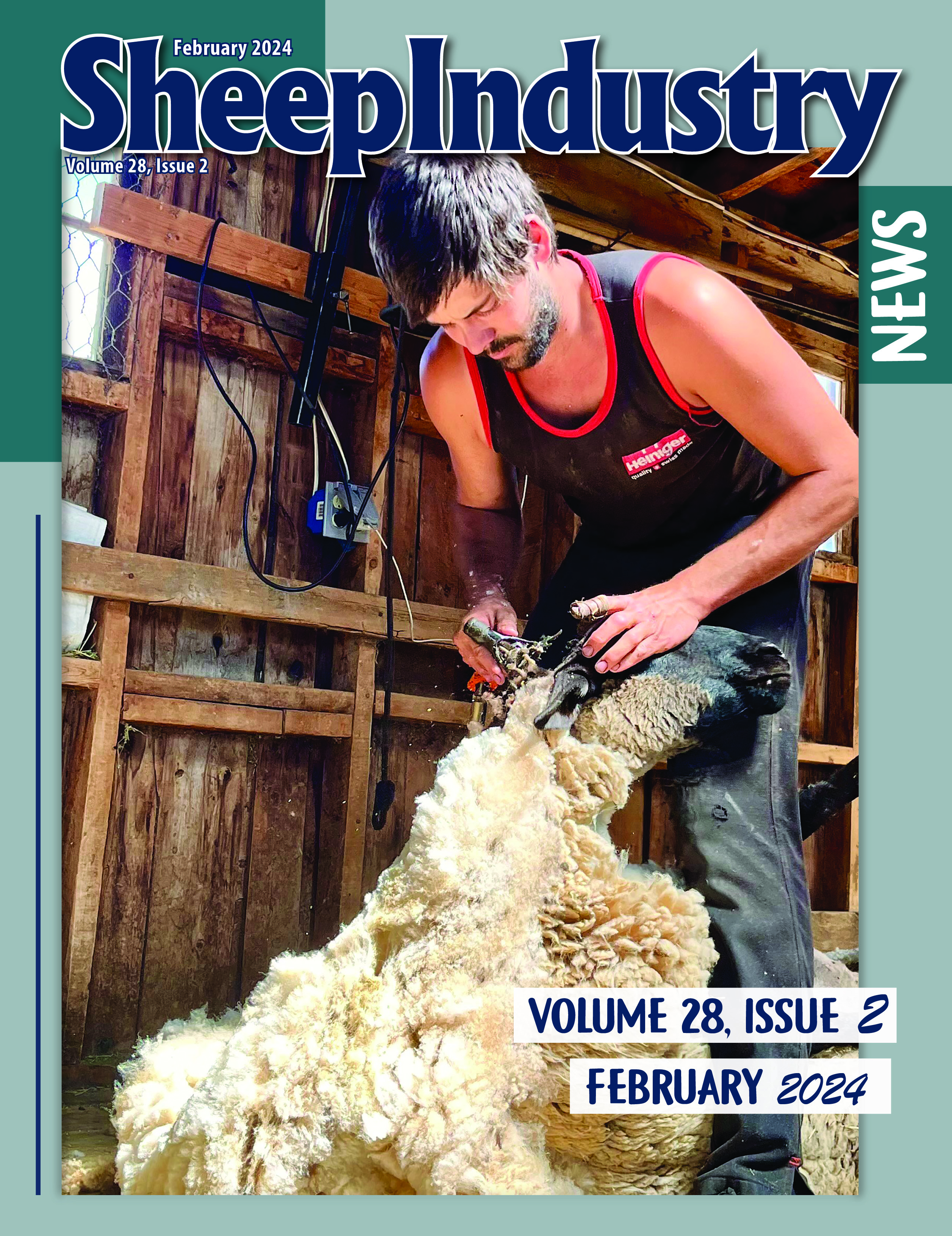The image is the cover of a magazine titled "Sheep Industry," framed by a greenish border. Across the top, in dark blue letters with white outlines, it says "Sheep Industry," with "February 2024" written in white above it. Below the main title, in smaller white text, it states "Volume 28 Issue 2." Both the lower right corner and the right side feature white banners with dark blue lettering, repeating "Volume 28 Issue 2" and "February 2024."

In the central image, a man with short dark hair, a beard, and a mustache is shearing a sheep. He wears a black tank top with red trim that has "Henninger" written in white and red, and blue jeans. The man holds a pair of electric shears in his right hand, while his left hand rests on the sheep, which is white with brown markings around its nose and ears. The sheep gently leans its head against the man's leg.

The scene is set inside a barn or stable with wooden walls, visible beams, an open window covered with chicken wire, and an electrical box filled with various plugs. The trimmer's white cord is seen connected to this outlet setup.